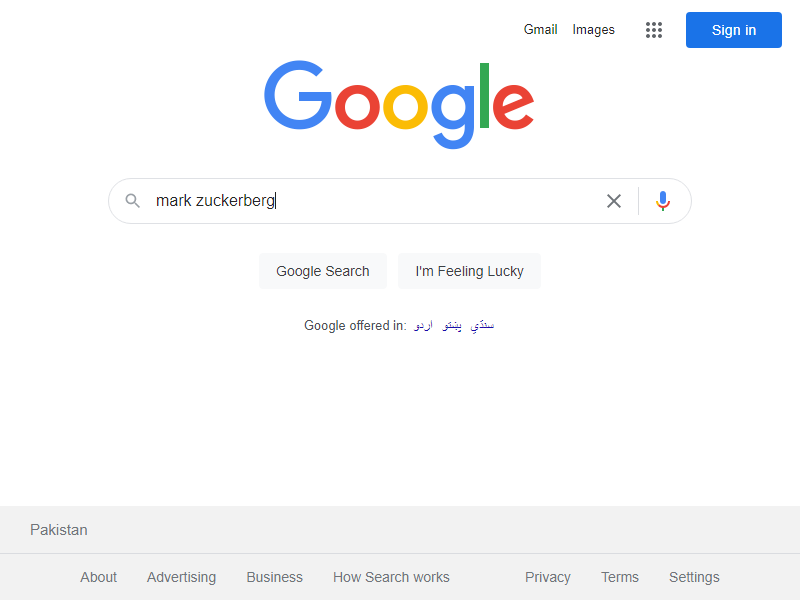A screenshot depicts the main Google search page with the name "Mark Zuckerberg" partially typed in the search bar, with the cursor blinking at the end of the name. The page is characterized by its signature clean, white background and the colorful Google logo consisting of the primary colors: blue, red, yellow, and green. Below the search bar, the familiar "Google Search" and "I'm Feeling Lucky" buttons are prominently displayed. The page shows that the user is not signed into their Google account, and language options include Farsi or Arabic, suggesting localization features. Additionally, a subtle hint in light grey at the bottom of the screen indicates the user's geographical location as Pakistan. No search results or images are displayed, as the search has not yet been executed.